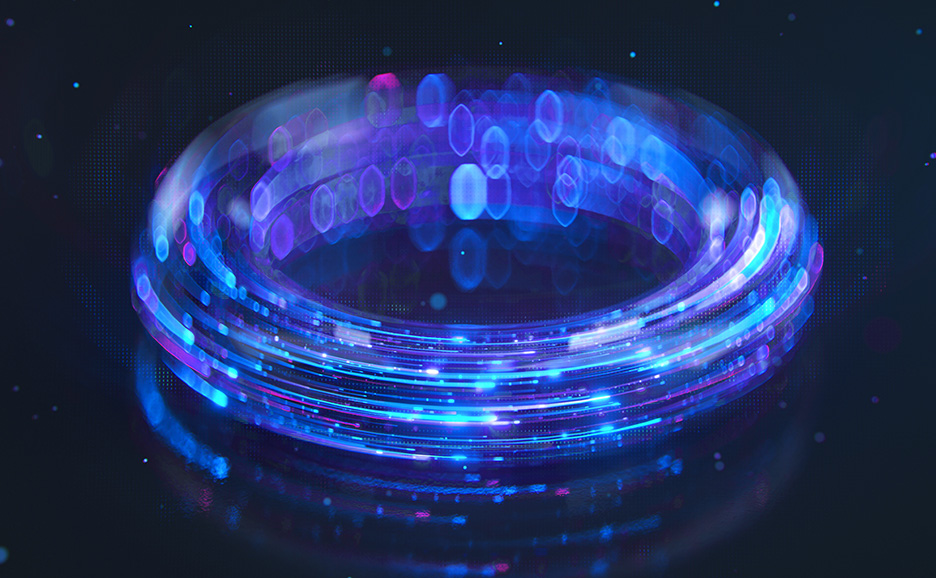The image depicts a captivating cosmic scene, featuring a vibrant, swirling ring of neon lights set against a deep black background adorned with tiny pixel-like dots, reminiscent of distant stars or digital pixels. The ring, resembling a delicate bracelet, is composed of multiple layers—approximately 40 to 50—of string-like lights in an array of colors including purples, blues, reds, whites, and magentas. These lights appear in motion, giving the impression of high-speed rotation or futuristic technology, evoking imagery akin to fast-moving data or light. The ring's swirling pattern and multicolored lights create a mesmerizing, tech-savvy visual against the blurred, abstract background, enhancing the dynamic and modern aesthetic of the image.